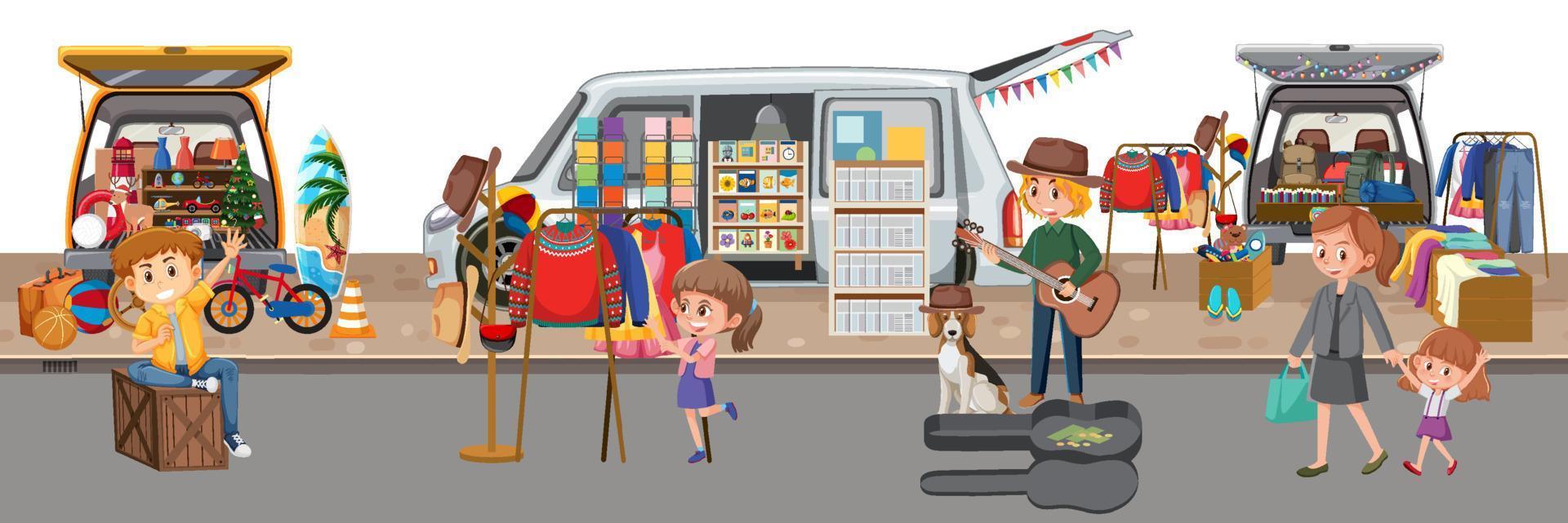This vibrant and detailed cartoon image depicts a lively street festival, where several people are selling various items from the trunks and sides of their vans. On the far left, a boy in a yellow jacket sits on a crate, waving with one hand. He is in front of a yellow van adorned with a variety of items such as bicycles, beach balls, a surfboard, a suitcase, and even a Christmas tree. The middle of the image features a girl in a purple dress, pink jacket, and purple shoes with her hair in a ponytail, selling clothes from racks filled with sweaters and hats. Behind her is a van decorated with a flag banner, which appears to be selling books and magazines. Next to her, a man with a green shirt and blue jeans strums a guitar while his dog, wearing a hat, sits beside him. His open guitar case, scattered with cash, sits on the sidewalk. On the right side of the image, a woman in black attire and black shoes carries a blue bag while holding the hand of a little girl in a pink overall dress and red shoes. They walk past another van that is selling various clothes and accessories displayed on racks and wooden stands. The entire scene is full of vibrant colors and whimsical details, capturing the bustling and festive atmosphere of a community market.